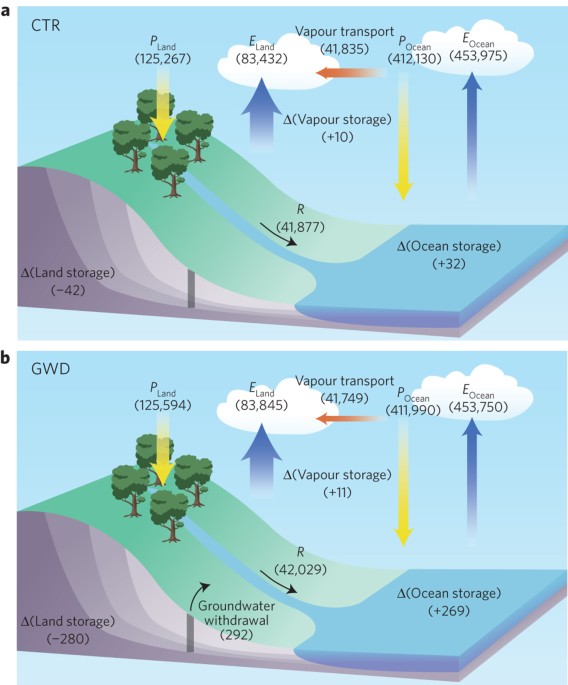The image comprises two diagrams, stacked vertically and labeled A (top) and B (bottom), elucidating the water cycle. Both diagrams feature a gently sloping hill adorned with trees and a stream flowing towards a blue body of water at the base, symbolizing the ocean. In the background of each image, light blue skies and white clouds float, maintaining a consistent atmospheric setting.

In Diagram A (top), labeled "CTR" in the upper left corner, several elements illustrate various stages of the water cycle with accompanying numerical data. A yellow arrow pointing downward through the trees represents precipitation on land (P_land = 125,267). An arrow marked "R" flows down the slope with the number 41,877, indicating runoff. Ocean storage, denoted by a Delta symbol (Δ), shows a positive change (+32). Vapor transport is marked by a red arrow moving towards the left cloud, labeled "ocean" (vapor transport = 41,835), while vapor storage features another Delta symbol (Δ, +10). The clouds in the background indicate different sources of evaporation: E_land, E_ocean, and P_ocean, each with different figures. There are multiple blue arrows pointing upwards, symbolizing evaporation processes, and at the bottom left of the hill, land storage is indicated with a negative value (Δ land storage = -42).

Diagram B (bottom), labeled "GWD" in the upper left corner, mirrors Diagram A in structure but features different numerical values and additional information. Notably, it includes "groundwater withdrawal" (292) beneath the hill, altering the water cycle dynamics by accounting for groundwater extraction.

This intricate depiction highlights the movement of water from land and ocean sources into the atmosphere, via evaporation and vapor transport, and its subsequent return through precipitation and runoff, differentiated by quantitative data and including the impact of groundwater withdrawal in Diagram B.